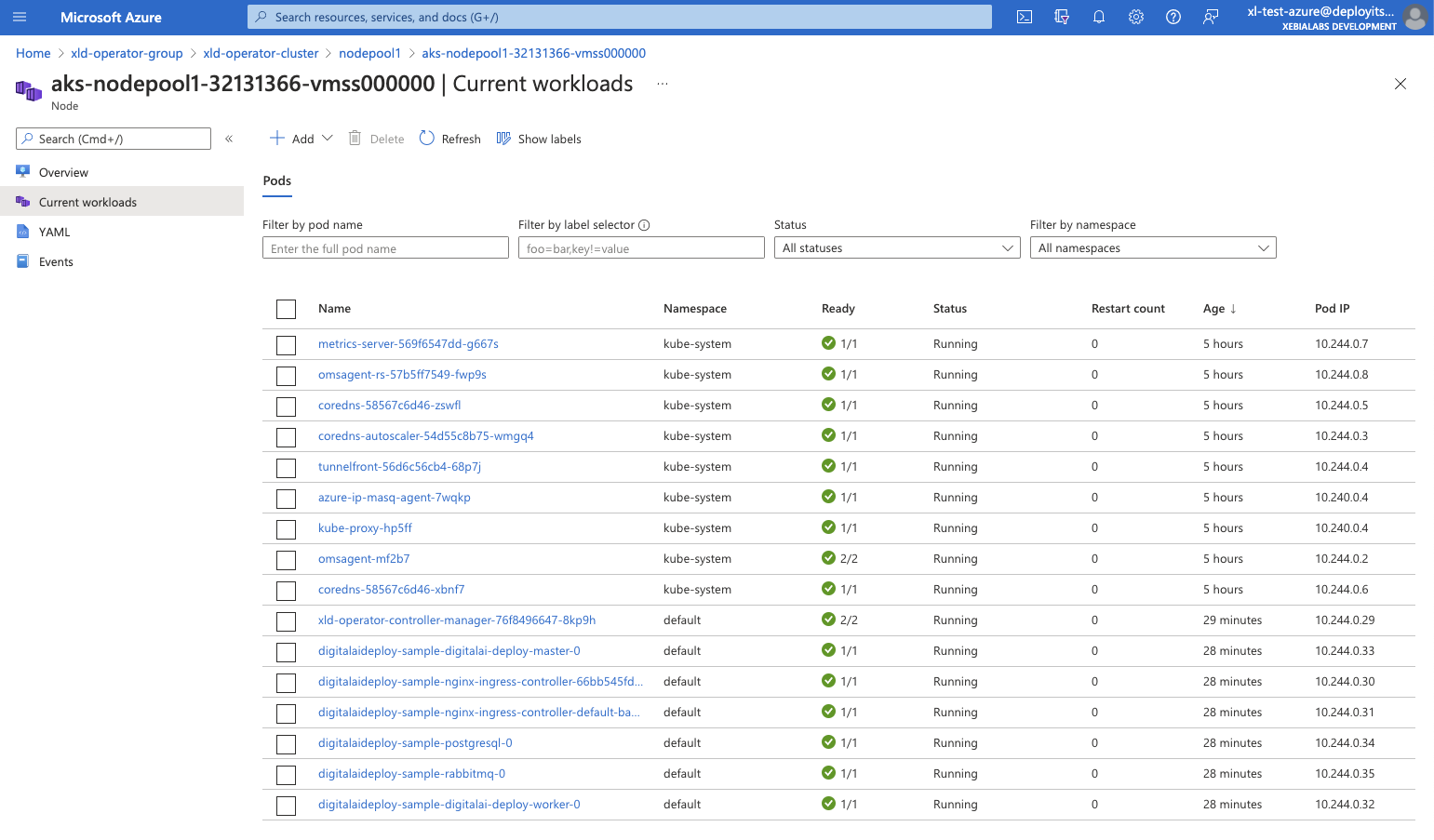This image is a detailed screenshot from the Microsoft Azure platform. At the very top, a prominent blue banner displays "Microsoft Azure" in crisp white text. Just below the banner is a long search bar with the placeholder text "Search resources, services, and docs," enabling users to quickly locate various features and documentation within Azure. To the right of the search bar, several interactive icons are lined up: a bell icon for notifications, a gear icon for settings, a question mark icon for help or FAQs, and the partially obscured email address of the current user, maintaining some privacy.

The main section of the interface is predominantly white and features an organized, spreadsheet-like layout. The hierarchical navigation path displayed indicates that the user is working within the following structure: Home > XLD Operator Group > XLD Operator Cluster > Node Pool One > AKS Node Pool One, each representing nested segments of the project.

Within the Current Workloads section, the display resembles a to-do list with each task entry outlined in rows. Each row includes a tickable checkbox on the left, allowing for task completion tracking. Following the checkbox, several essential columns are clearly labeled: Name, Namespace, Readiness, Status, Restart Count, Age, and Pod IP. These columns provide a comprehensive overview of each entry, facilitating efficient management and monitoring of workloads.